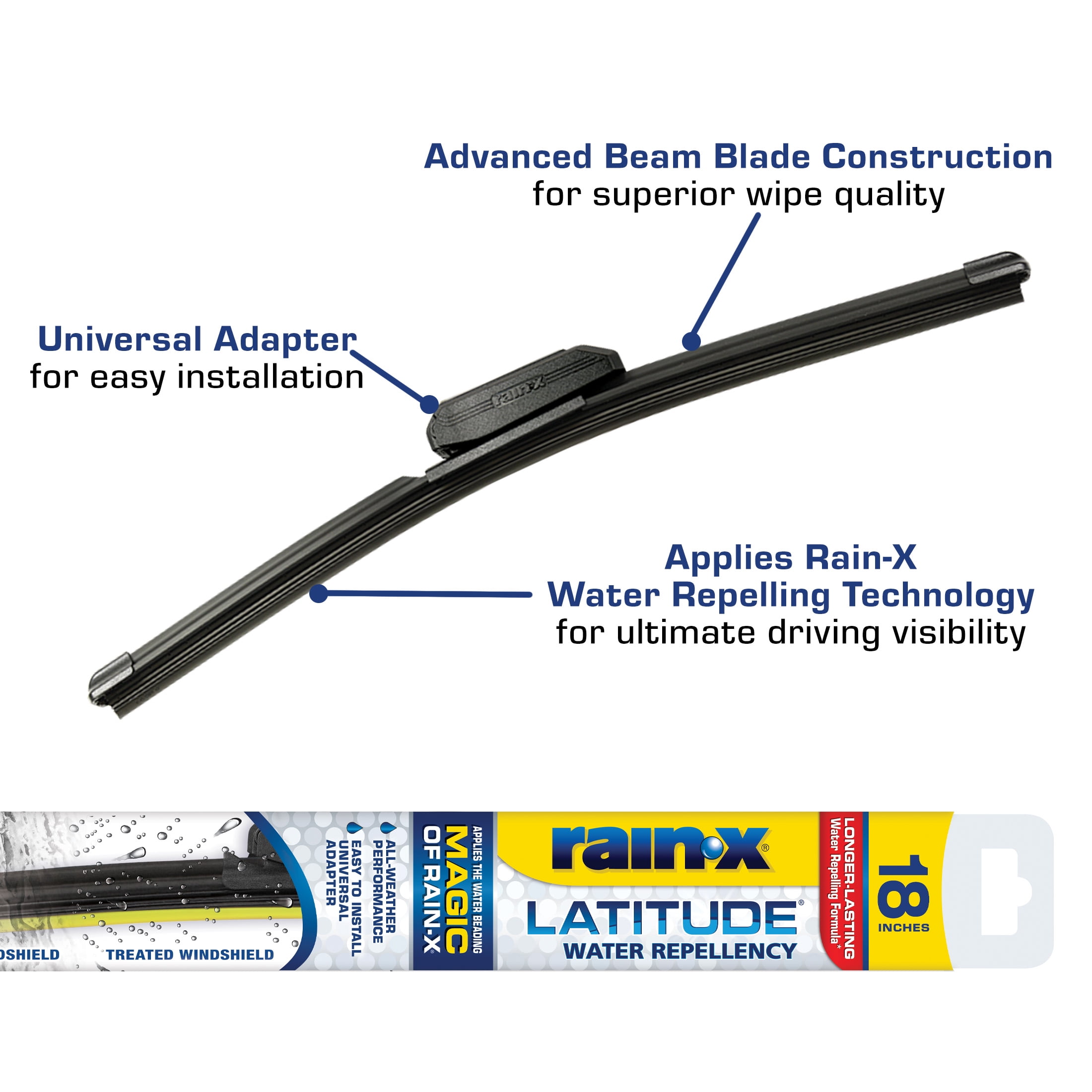The image is an informational graphic for the Rain-X Latitude Water Repellency windshield wipers, specifically highlighting an 18-inch model. The prominently displayed text emphasizes key features such as "Advanced Beam Blade Construction for Superior Wipe Quality" and "Water Repelling Technology for Ultimate Driving Visibility." The graphic details a universal adapter for easy installation, showcasing advanced beam blade construction for quality wiping performance in all weather conditions. The wiper blades feature a longer-lasting water-repelling formula that applies the renowned Rain-X water-beading effect. The text, presented in a mix of navy blue for headings and black for detailed descriptions, notes these wipers provide enhanced driving visibility and all-weather performance. Additionally, the packaging is depicted with a white, yellow, and blue color scheme, illustrating the product's design and branding.